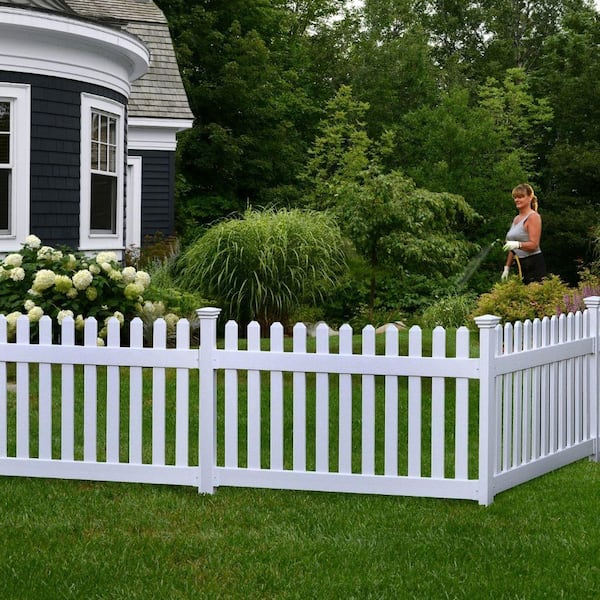The image depicts a serene backyard of a residential home surrounded by an inviting and well-maintained green lawn. Dominating the foreground is a woman with blonde hair pulled back in a ponytail, wearing a gray tank top and black pants, who is attentively watering plants using a hose with a nozzle. The backyard is enclosed by a charming white picket fence and features a variety of plants, including tall, grassy foliage and a significant bush adorned with large, white, bulbous flowers. The backdrop reveals several towering trees that create a forested effect, enhancing the tranquil atmosphere. The house itself has a cottage style with a very dark gray, wooden exterior, complemented by white window sills and trim, leading up to a gray roof with a distinct dome-style structure. The setting suggests a peaceful moment in either early morning or late afternoon, highlighting the harmonious blend of nature and homely comfort.